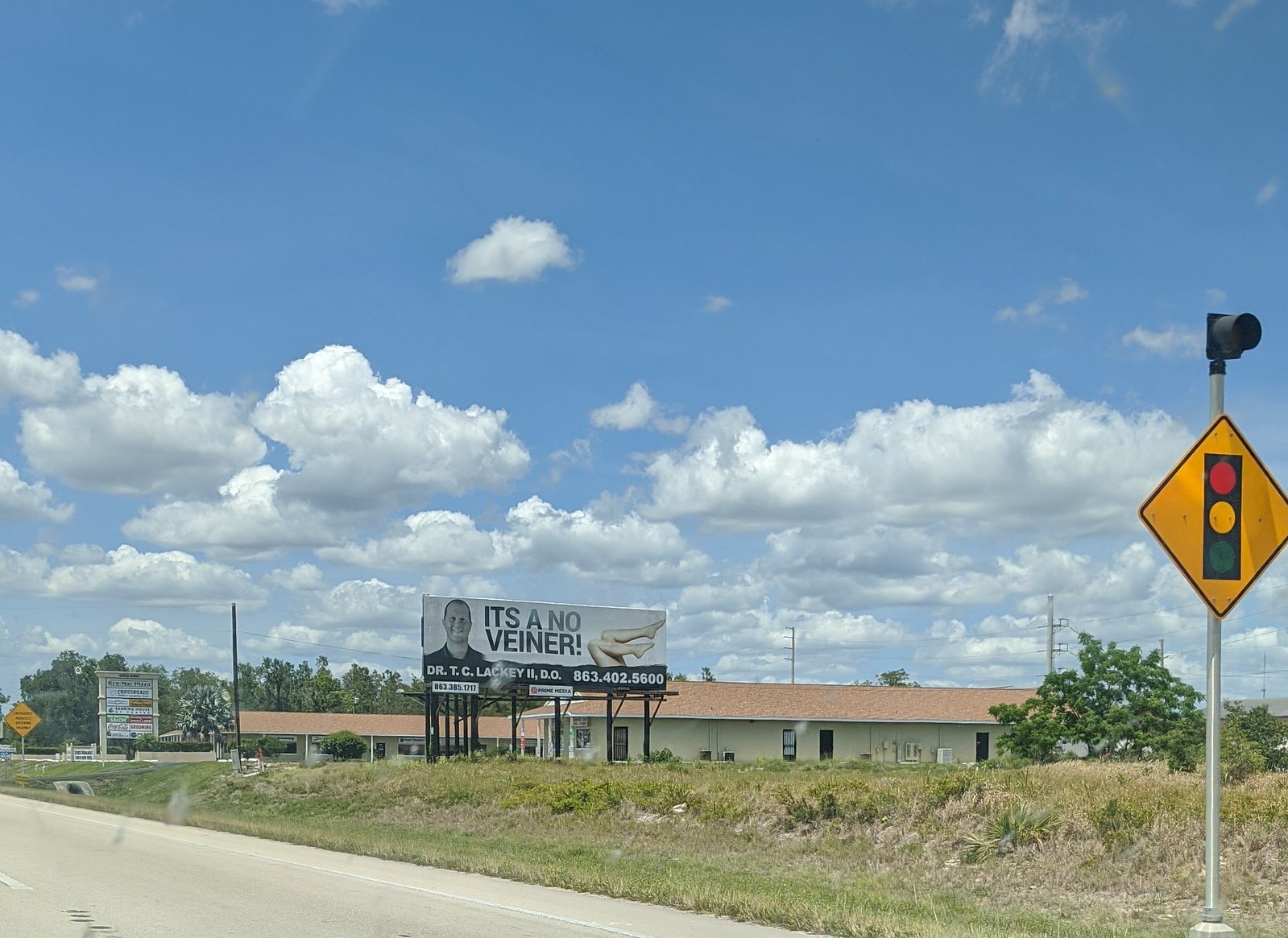The image depicts a rural outdoor scene captured on a bright, sunny day, with clear blue skies adorned with puffy white cumulus clouds stretching to the horizon. Dominating the center of the image is a prominent billboard mounted on a dark scaffolding structure, advertising vein care services with the slogan "It's a no-veiner!" It features a pair of woman’s legs raised in the air and a smiling portrait of Dr. T.C. Lackey, DO, accompanied by a contact phone number. The billboard stands in front of a building that appears to be a light yellow convenience store with a brown asphalt shingle roof.

The surroundings include a slight grassy berm with patches of dead grass and a low, scrubby tree. To the right side of the image, a yellow diamond-shaped warning sign on a silver aluminum pole indicates an upcoming traffic signal. Further down the road, another business sign and a caution sign are visible. The scene suggests a setting adjacent to a main road, likely a highway, flanked by a grassy expanse and marked by signal signs hinting at a remote, rural location.